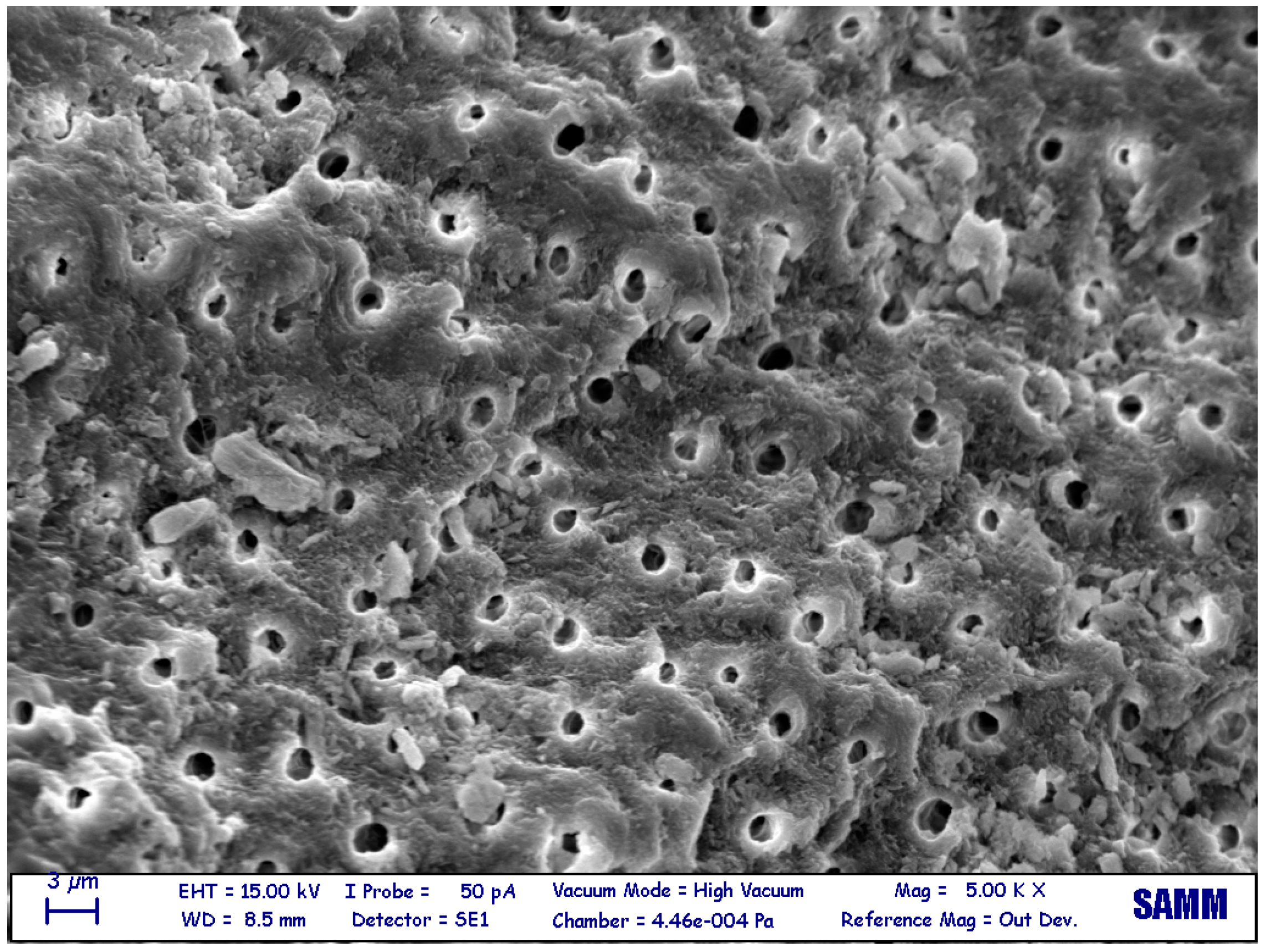The image depicts a highly magnified, black-and-white photograph likely taken through a microscope. The central subject is a gray-colored coral-like structure featuring numerous black dots. This microscopic view reveals intricate details of the mass, which includes small holes or pores. Surrounding the primary image, at the bottom right corner, is a white rectangular overlay that contains various pieces of technical information presented in navy blue text. Key details include "SAMM" and "3UM," which most likely denote the scale (3 micrometers). Additional technical specifications are provided, such as "EHT = 15.00 kV," "WD = 8.5 mm," "I-probe = 50 PA," "detector = SE1," and "vacuum mode = high vacuum." The chamber pressure is listed as "4.46 E-004 PA," and the magnification is "5.00 kx," with a reference magnification labeled "outdev." This contextual information, placed against a white background, aids in understanding the microscopic scale and conditions under which the image was captured.